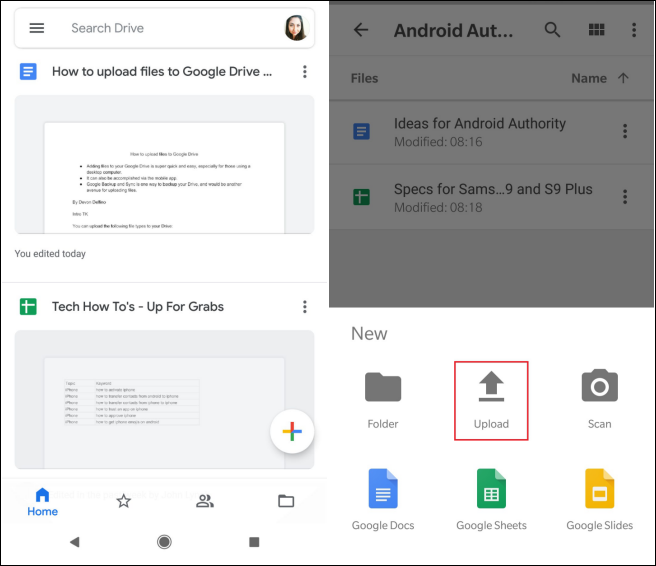This image is a detailed screenshot showcasing two distinct user interfaces side-by-side.

**Left Panel: Google Drive Interface**
- **Header**: At the top, there is a search bar with light gray boundaries and a white center. The left side of the search bar features three horizontal lines, the middle displays the gray text "Search Drive," and the right side contains a circular avatar of a young female user with black hair.
- **Content**: 
  - Below the search bar, a blue Google Docs icon precedes the text "How to Upload Files to Google Drive," followed by three vertical dots indicating further options.
  - Underneath, a rectangular snippet of a Google document with a light gray background partially displays text, including a blurred title "How to Upload Links to Google Docs," three visible bullet points, and brief lines of text. The document is marked as edited today.
  - A thin dividing gray line separates this from another section featuring the Google Sheets icon next to the title "Tech How To's - up for grabs," followed by another set of three vertical dots. Below this, a grayed-out preview of a Google Sheets page includes a plus symbol button to create a new Google Sheet in the bottom right corner.
- **Bottom Navigation**: At the very bottom of the page, four icons are aligned:
  - A blue "Home" icon with a house symbol indicating the current selection.
  - An unselected open star icon.
  - An icon representing two overlapping user figures.
  - A folder icon.
- **Playback Controls**: Along the bottom edge are three additional icons:
  - A left-facing triangle.
  - A gray recording button.
  - A gray stop button.

**Right Panel: Android Authority Files Interface**
- **Header**: The upper section features a dark gray background with a left-facing arrow, the truncated text "Android Auth...," a search magnifying glass, a 2x3 grid of squares, and three horizontal dots.
- **Main Content**:
  - A dividing line separates the header from the file listing below.
  - The section headers include "Files" on the left and "Name" with an upward-facing arrow on the right.
  - Two files are listed:
    - A Google Doc named "Ideas for Android Authority," modified at 08:16.
    - A Google Sheet named "Specs for SAMS 9 and S9+," modified at 08:18.
- **Bottom Section**: The lower part of the panel displays a grid layout titled "New" in the upper left. The grid comprises six app icons arranged in a 2x3 format:
  - A folder icon labeled "Folder."
  - An upload icon with a red square background.
  - A scan icon with a camera.
  - Google Docs icon.
  - Google Sheets icon.
  - Google Slides icon with a yellow background in the bottom right corner.

This detailed screenshot efficiently captures the structure and elements of both the Google Drive search interface and the Android Authority file management interface.